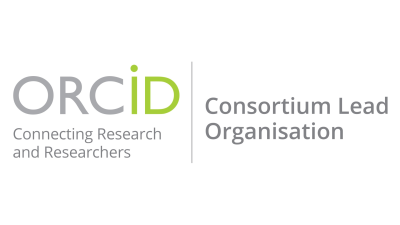The image features a purely text-based design on a white background, devoid of any photographic or illustrated elements. On the left side, prominently displayed are the words "ORC ID," with "ORC" in capital letters in dark gray and "ID" in a vibrant neon green, where the "I" is lowercase and the "D" is uppercase. Directly below this, in a smaller, subdued gray font, is the phrase "Connecting Research and Researchers." A thin gray vertical line separates this section from the text on the right. On the right side of this vertical line, the phrase "Consortium Lead Organisation" is displayed in gray letters, with "Organisation" notably spelled with an 'S' instead of a 'Z'. The entire composition is straightforward and clean, emphasizing the text without any additional elements such as people, animals, plants, or vehicles.